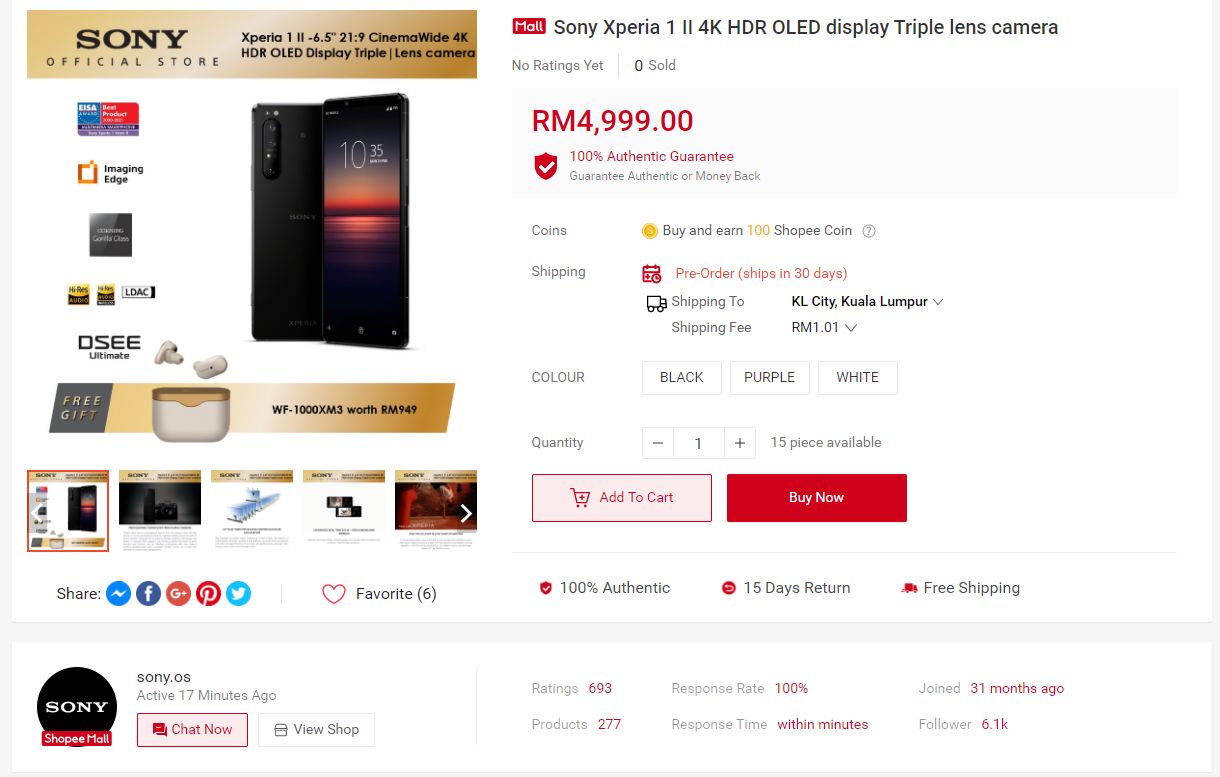**Product Description: Sony Xperia 1 II - 6.5-inch Display, 21:9 CinemaWide 4K HDR, Triple Lens Camera**

**Overview:**
Introducing the Sony Xperia 1 II, an official Sony product, equipped with a 6.5-inch 21:9 CinemaWide 4K HDR display. This smartphone boasts a remarkable triple lens camera setup, ensuring professional-grade photography and videography.

**Key Features:**
1. **Display:** The Xperia 1 II features a stunning 6.5-inch 21:9 CinemaWide 4K HDR display, providing an unparalleled visual experience.
2. **Camera System:** Triple lens camera system for versatile and high-quality photography.
3. **Audio Quality:** High-resolution audio and LDAC support for an ultimate listening experience.
4. **Additional Features:** Includes a free gift - the WF-1000XM3 wireless noise-canceling earphones (worth RM949).

**Pricing and Availability:**
- **Price:** RM 4999.00
- **Color Options:** Black, Purple, White
- **Available Stock:** 15 pieces
- **Quantity Selection:** Options to add or reduce quantity before adding to cart.
  
**Purchase and Shipping Details:**
- Earn 100 shopping coins with each purchase.
- Shipping to Kuala Lumpur (KL) with a minimal fee of RM 1.01.
- Order ships within 30 days.
- Free shipping for returns.

**Seller Information:**
- **Seller:** Trippin, highly rated with a 100% content guarantee.
- **Response Rate:** 100%
- **Active Time:** 17 minutes ago
- **Membership Duration:** Joined three months ago
- **Rating:** 693
  
**Additional Information:**
- Shareable on social media platforms like Facebook, Messenger, Google Plus, Pinterest, and Twitter.
- The product listing is authenticated and comes with a money-back guarantee.

Experience cutting-edge mobile technology with the Sony Xperia 1 II, combining premium visuals, audio, and photography in one sleek device. Add to cart or buy now to elevate your tech game.